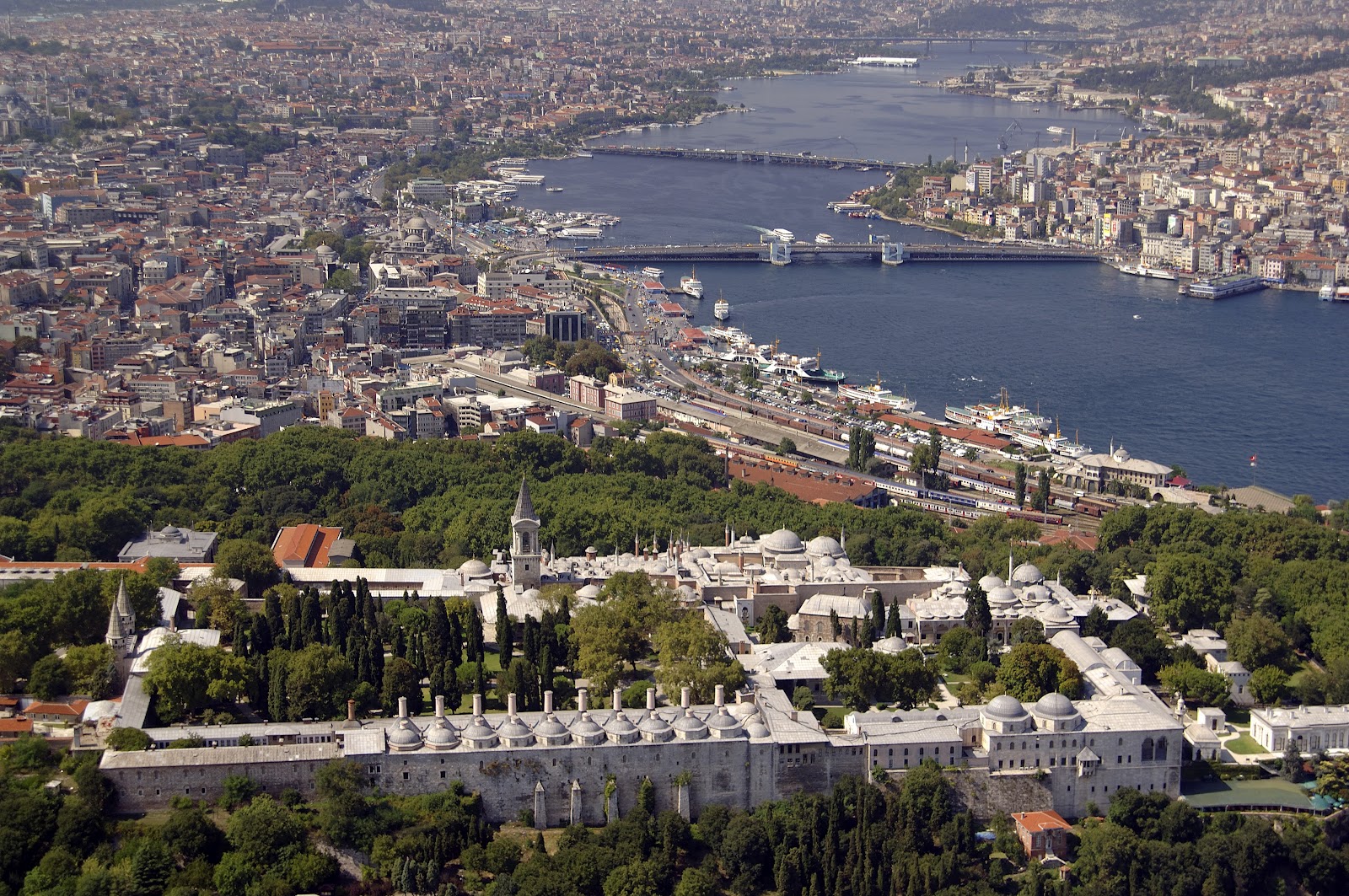This is a detailed aerial view of a sprawling city intersected by a large river that flows in from the top right and curves through, exiting the image to the right. The bustling urban landscape is dominated by numerous buildings on either side of the river, with three prominent bridges connecting both sides. A railroad with a visible train adds to the city's intricate infrastructure. In the lower portion of the image, there is a low, rectangular white building, possibly a palace or government structure, characterized by its ornate steeples, domes, and a square central courtyard. This notable building is surrounded by dark green trees, providing a stark contrast to the densely populated cityscape dominated by tan and beige structures. The area around this building includes a central garden, highlighting a pocket of greenery in an otherwise highly urbanized environment.